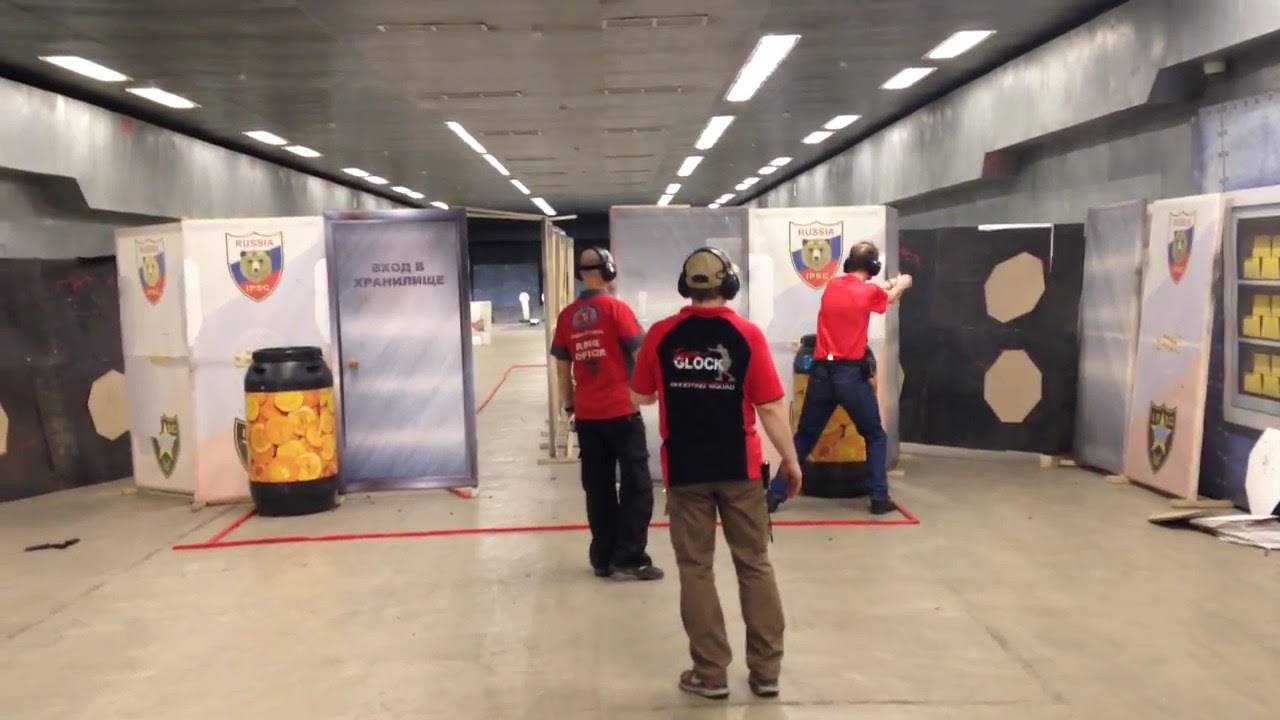The image captures an indoor firing range with a deep, warehouse-like room featuring a low roof and a beige, gymnasium-like floor. Towards the center, three men stand in red shirts, equipped with ear protection. One of the men is actively shooting at targets that are strategically placed throughout the room. The targets and dividers, resembling elements of an obstacle course, include makeshift objects like doors and barrels. Symbols and text, possibly in an Eastern European language, are visible on the targets—one notable emblem includes “Russia IPSC” along with a bear in a shield. The setting is vivid with colors like tan, red, yellow, blue, and various shades of gray and dark blue, contributing to the detailed scene of a specialized training environment.